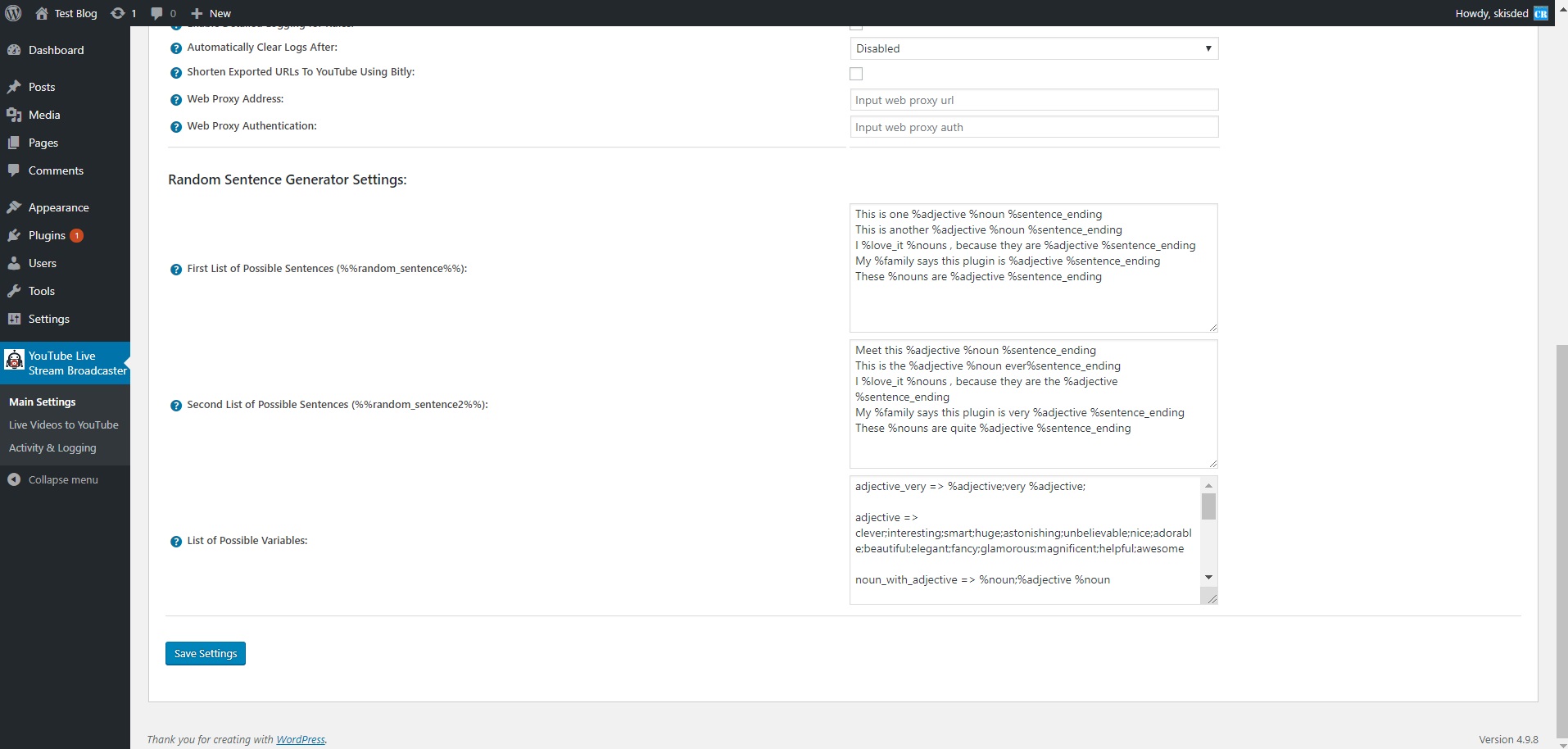Screenshot of a WordPress Dashboard Featuring a YouTube Live Section

This detailed image displays a WordPress dashboard with an additional YouTube live section, suggesting the use of a specialized extension. The dashboard presents multiple navigation rows on the left, including Dashboard, Posts, Media, Pages, Comments, Appearance, Plugins, Users, Tools, and Settings. The YouTube live section, currently selected, reveals an array of settings on the right side.

In this YouTube live extension, users can find options like automatically clearing logs after a specified time, shortening exported URLs to YouTube using bit.ly, and toggling the web proxy address on or off. The interface provides fields for entering the web proxy address and web proxy authentication. There are also text boxes dedicated to random sentence generation, allowing users to input the first line of potential sentences, a second line, and a list of possible variables.

At the bottom left of this section, a prominent blue button enables users to save their settings. On the top right, a partially blurred welcome message reads "Howdy," with the user's name obscured for privacy. The background across most of the interface is white, contrasted by a dark grayish-blue panel at the top and left side, giving a clear and organized appearance to the dashboard.